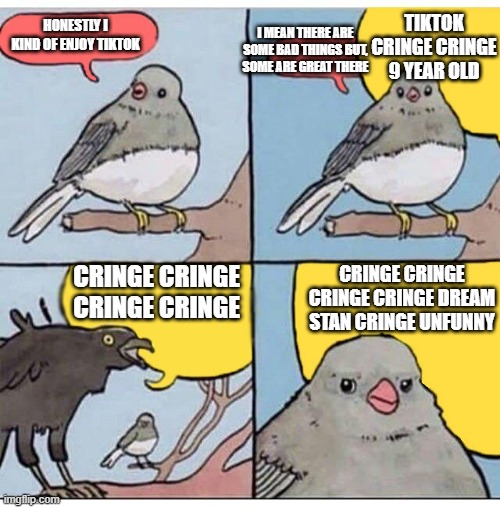**Image Caption:**

The artwork is divided into four panels, arranged in a 2x2 grid separated by a black bar. Each panel appears to be a hand-drawn, possibly watercolor illustration depicting an inn. 

In the upper-left panel with a blue background, a light brown tree trunk rises from the bottom right corner, culminating in a small branch extending to the left. Perched on the branch is a pigeon, gray on top with a white underside. A red speech bubble to the left of the pigeon contains white text that reads, "Honestly, I kind of enjoy TikTok."

The upper-right panel replicates the scene on the left, but the pigeon is now looking directly at the viewer. The red speech bubble features the text, "I mean, there are some bad things, but some are great."

In the lower-left panel, the perspective pulls out to show the entire setting. A large black raven dominates the foreground on the left-hand side, with a yellow speech bubble containing the word "cringe" repeated three times in white.

The lower-right panel zooms in on the same pigeon from the previous panels. The pigeon, now looking furious, is accompanied by a yellow speech bubble that repeats the words "cringe," "cringe," "cringe," followed by "dream stand," "cringe," and "unfunny."

The image delivers a commentary on mixed feelings towards TikTok, illustrating the divided opinions about the platform's content.